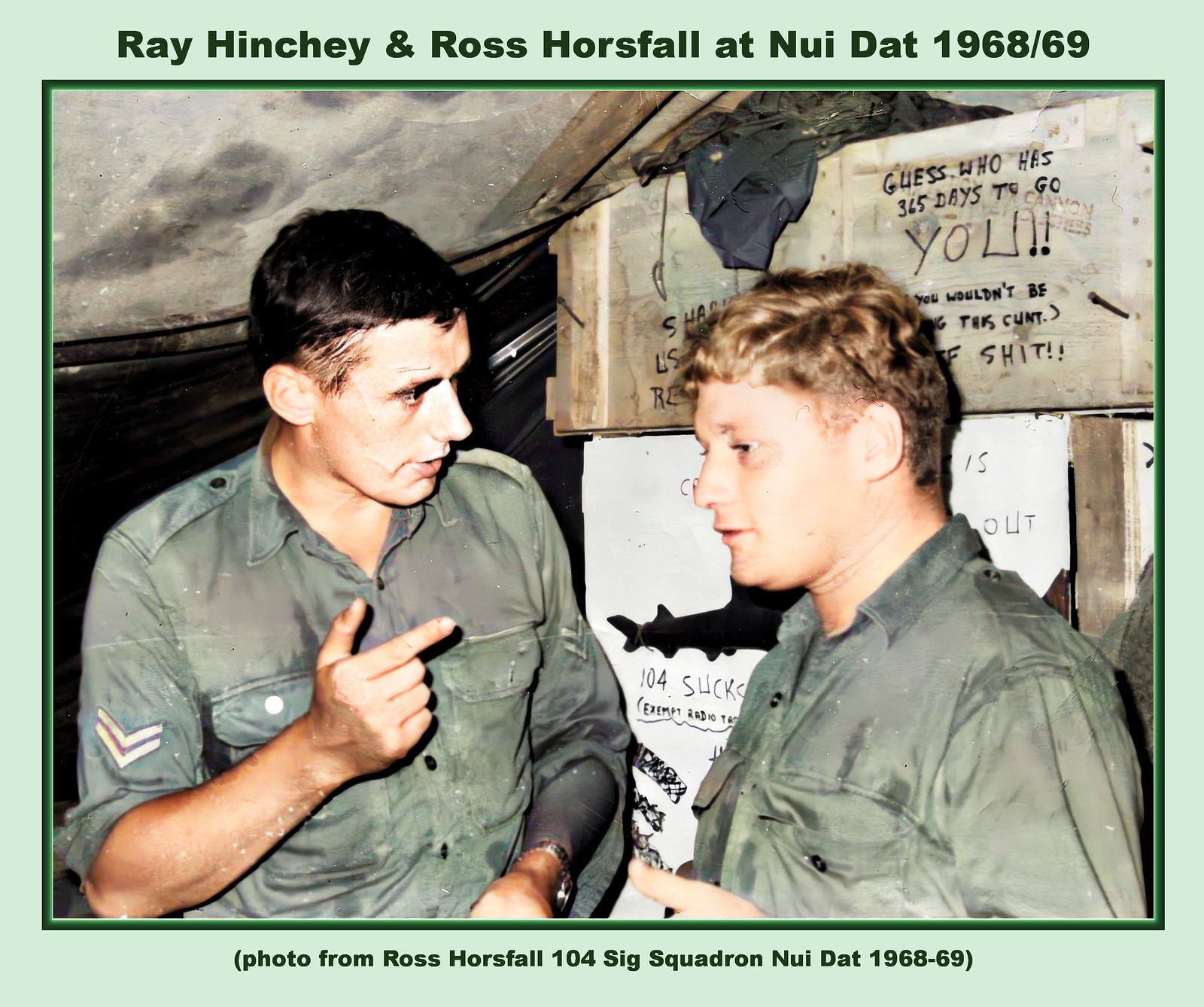In this photograph, two men dressed in green military uniforms are seen standing in a sheltered structure in front of crates and boxes, with the image captured from their waist up. The man on the right has short blonde hair, while the man on the left has short black hair and is wearing a watch. The man on the left, identified by two stripes on his sleeve, is gesticulating with his right hand, appearing to explain something to the man on the right. Both men are Caucasian and facing mostly towards each other. Above them, text reads, "Ray Hinchey and Ross Horsfall at Nui Dat, 1968-69," while below the photo, text states, "Photo from Ross Horsfall, 104 Sig Squadron, Nui Dat, 1968-69." Additionally, a sign in the background features an incomplete and expletive phrase, reading, "guess who has 365 days to go? You! You wouldn't be..." The image is bordered by mint green detailing, adding to its archival feel.